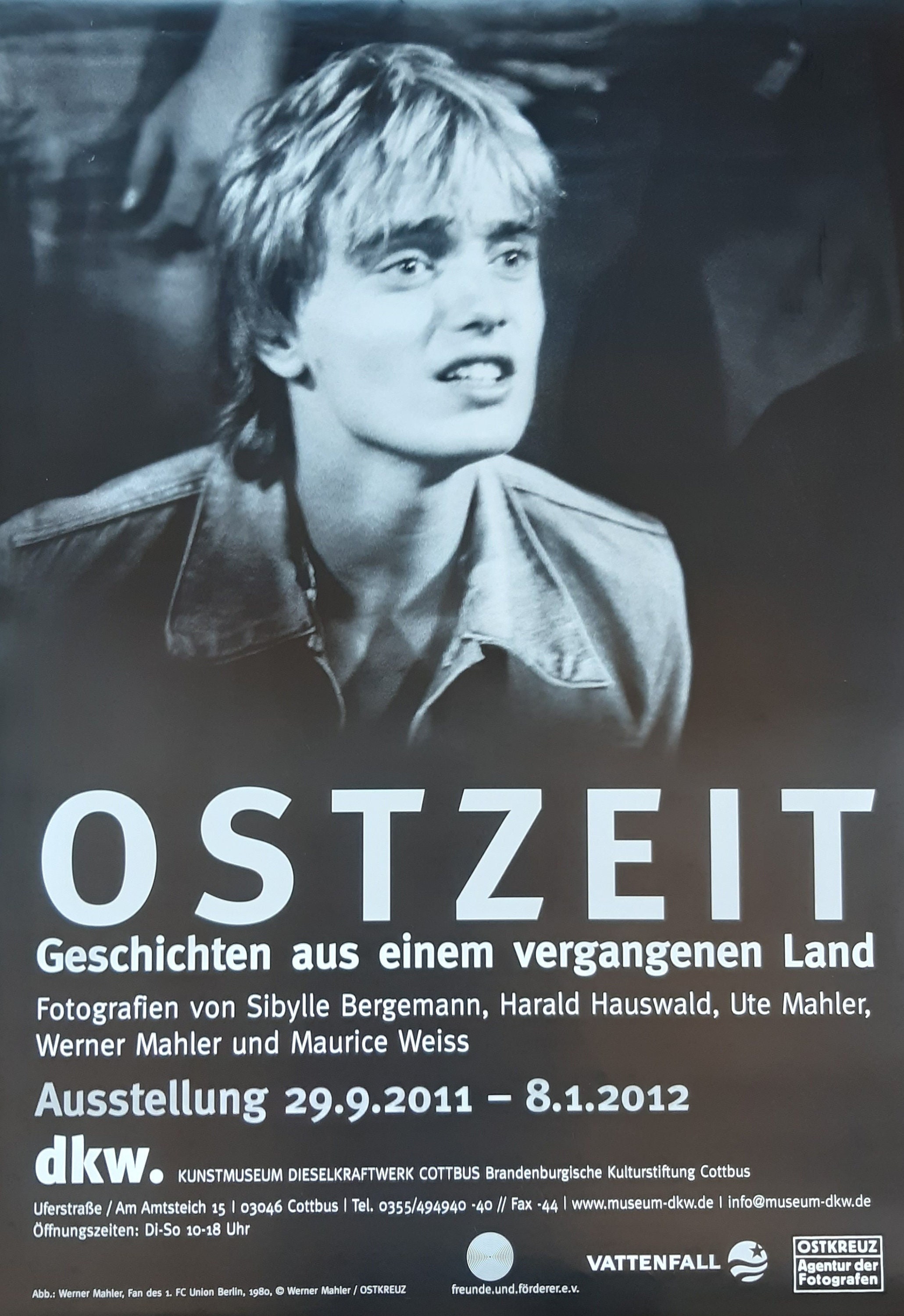A vertical poster features a black-and-white tinted image of a young blonde-haired man who appears to be either passionate or in distress. He has an androgynous appearance with a square jaw, plump lips, and twinkling eyes, sporting a mullet with bangs. His mouth is slightly open, revealing his front teeth, and he is dressed in a collared denim-like shirt. Behind him, other people are visible from their midriffs down, adding depth to the scene. The man is leaning forward and facing right. The lower part of the poster has bold white text on a dark gray background, reading "OSTZEIT." Directly below this, in smaller letters, it reads "Auszeitgeschichten aus einem vergangenen Land," which is German. The dates "September 29th, 2011 to August 1st, 2012" and the location "Kunstmuseum Dieselkraftwerk" are also listed. The poster seems to relate to the Berlin Wall, with various additional German words and logos at the bottom.